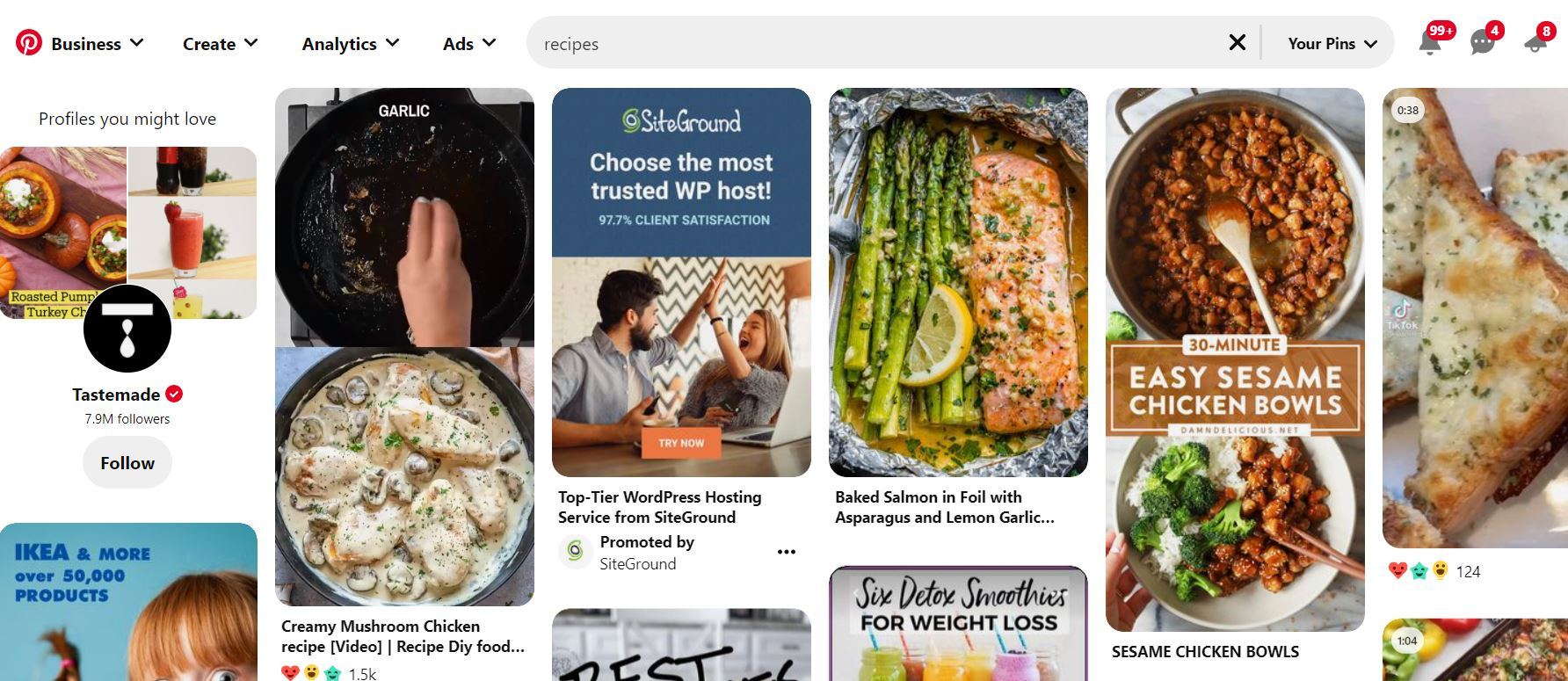This digital image showcases a Pinterest interface. In the top left corner, the Pinterest logo is prominently displayed. Just to the right, there is a navigation bar with tabs labeled "Business," "Create," "Analytics," and "Ads." Directly below these tabs is a search bar where the word "recipes" has been entered. In the top right section, there are notifications marked by a bell icon with the number 99 indicating unopened alerts. Adjacent to it is the message icon, accompanied by the number 4 showing unread messages.

The main content of the image features several enticing food pictures. One image depicts baked salmon wrapped in foil, accompanied by asparagus and lemon garlic, embodying a healthy dish. Another image showcases a "30 Minute Easy Sesame Chicken Bowls" recipe, featuring seasoned chicken in sauce with a spoon resting inside the dish. There is also a picture of golden, crispy garlic bread. Additionally, a creamy mushroom chicken recipe is presented, showing a bowl of chicken submerged in a rich, soup-like consistency. Each dish is visually appealing and invites the viewer to consider trying the recipes.